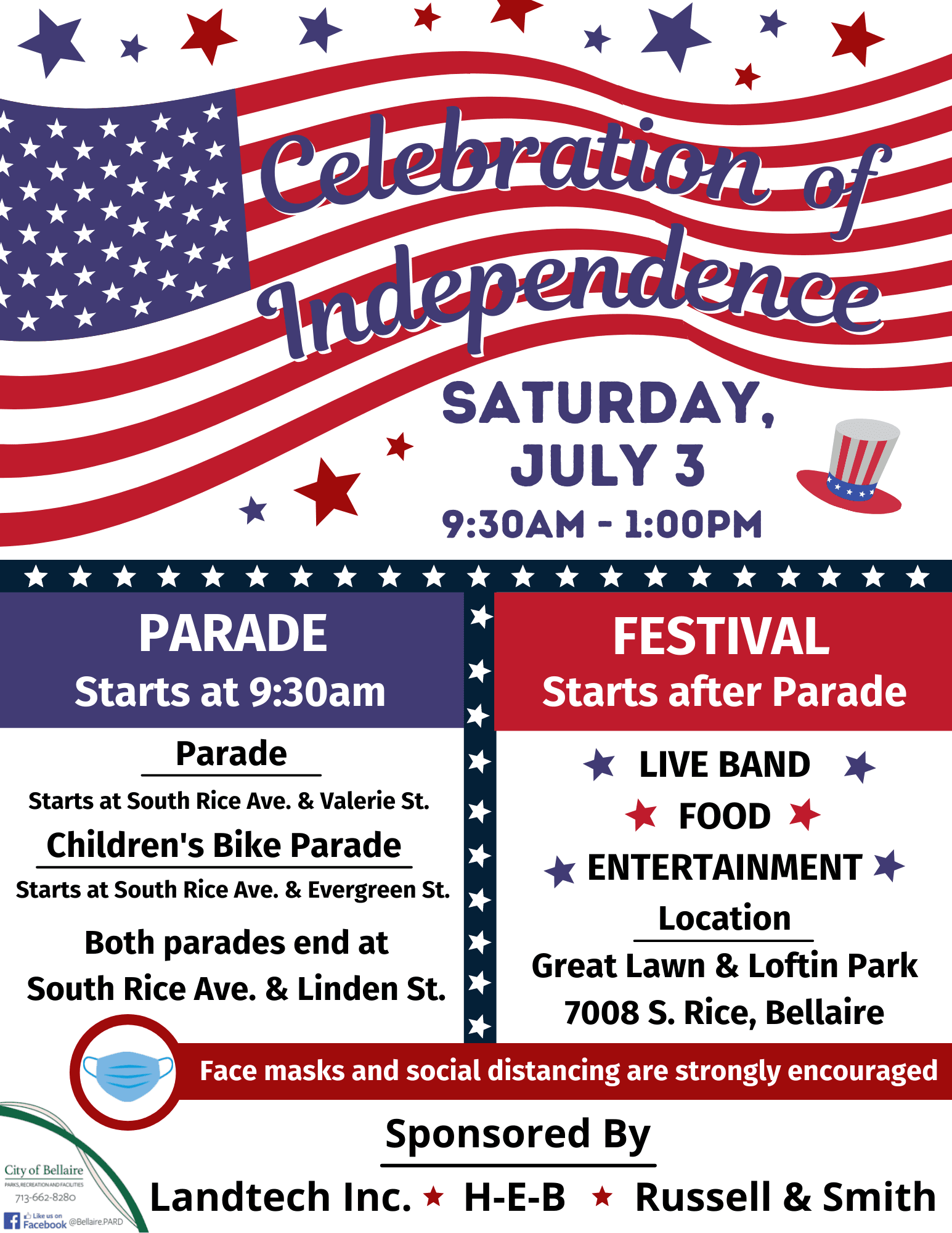Experience the "Celebration of Independence" on Saturday, July 3rd, from 9:30 a.m. to 1 p.m. This festive poster features a proud display of patriotism with a grand American flag, red, white, and blue stars scattered on a white background, and an iconic drawing of Uncle Sam's hat.

The event kicks off with a parade at 9:30 a.m. The main parade begins at South Rice Avenue and Valerie Street, while the children's bike parade starts at South Rice Avenue and Evergreen Street. Both parades will conclude at South Rice Avenue and Linden Street. This information is elegantly presented in white text on a blue background.

Following the parade, the festival will commence with live bands, delicious food, and entertaining activities for the entire family, located at the Great Lawn in Lofton Park, 7008 South Rice, Bel Air. The festival details are highlighted in white text on a red background, accentuated with blue and red stars.

In light of health protocols, face masks and social distancing are strongly encouraged, as indicated by a red strip featuring a blue mask symbol and corresponding text. 

The event is generously sponsored by Lantec Inc., H-E-B, and Russell and Smith. Additional highlights include a Facebook logo urging attendees to follow the City of Bel Air for updates and more information. Join us for a day of celebration, community, and American pride!